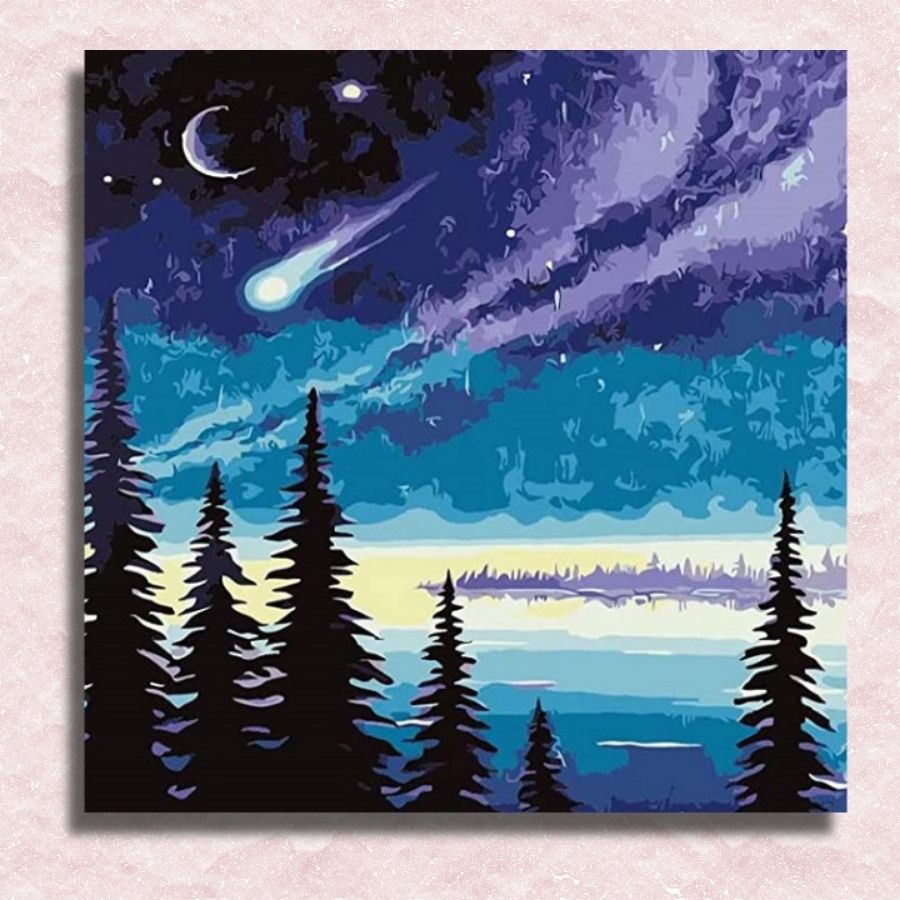Displayed against a textured, pale pink wall, this captivating canvas painting showcases a mesmerizing night sky within a dense forest scene. Dominated by cool shades, the artwork reveals the silhouettes of tall, dark pine trees standing in the foreground, while a serene lake or river captures light and transitions with a gradient of blue, subtly shifting into hints of yellow.

Above the tranquil waters, the detailed sky stretches across the upper half, painted in rich purples and deep blues. A prominent feature is the strikingly large, icy blue comet with a vibrant blue and purple tail streaking diagonally across the scene, illuminating the night with celestial beauty. The crescent moon hangs delicately to the upper left, accompanying three stars scattered across the sky. Furthermore, rolling hills with dark and lighter blue tones form a distant backdrop, completing this layered, enchanting nocturnal vista.